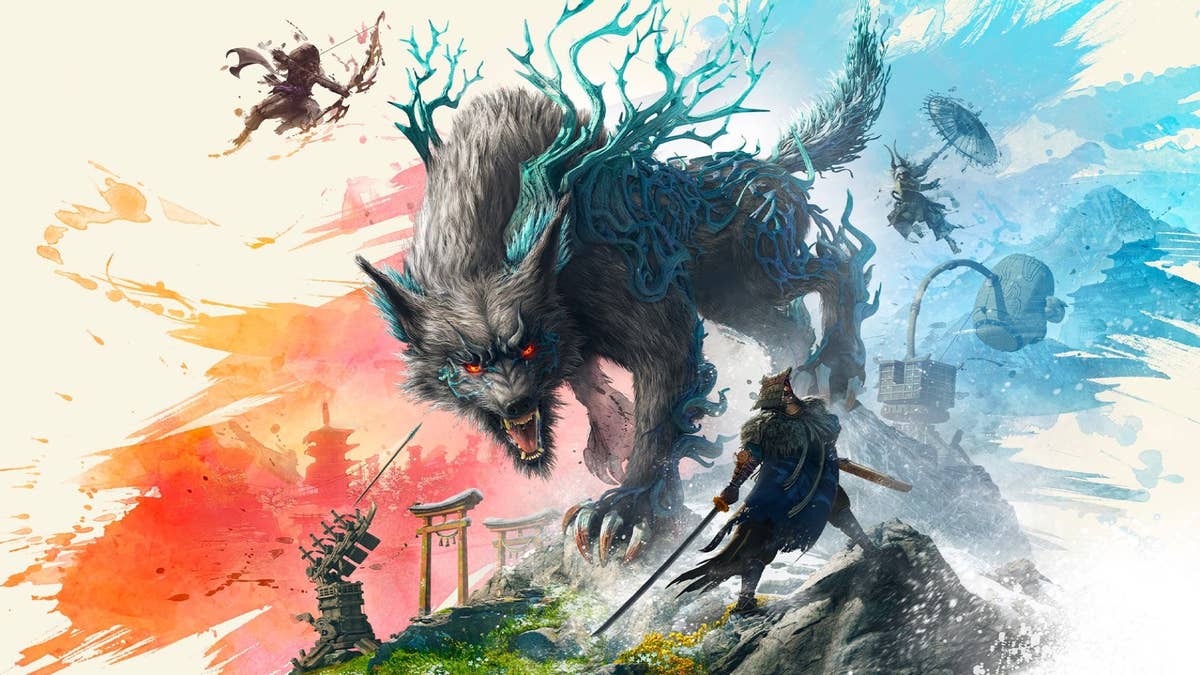The image is a highly detailed and colorful digital painting, depicting an epic scene of chaos and combat. At the center of the image is an enormous, terrifying werewolf-like creature with dense gray fur, blood-colored claws, and piercing red eyes. Its mouth is open wide in a fierce roar. Sprouting from its shoulders and tail are intricate, twisting, turquoise, root-like branches reaching skyward.

Surrounding the giant werewolf is a tumultuous battleground. Various warriors are engaging the beast: one with a sword, another with a bow, and a striking figure adorned in a blue robe wielding a katana. This robed warrior stands prominently on a rocky outcrop, his left hand extending the sword outward while his right hand holds a finely curved blade, possibly traditional like a katana. Adding to the surreal nature of the scene, a witch-like figure flies behind the werewolf holding an open umbrella, and another figure holding a parasol hovers mid-air, contributing to the chaotic tableau.

In the background, East Asian architectural elements, including Japanese archways with their distinctive curved tops and crossbars, are faintly visible. The landscape alternates between mountainous regions and vibrant, explosive colors— with splashes of pink, orange on the left, and bright blue teal on the right, blending into a dreamy, yet menacing atmosphere. Scattered machinery, including a hammer and spears, further intensify the scene's action. The piece collectively forms a vibrant tapestry of battle, magic, and mythic grandeur.